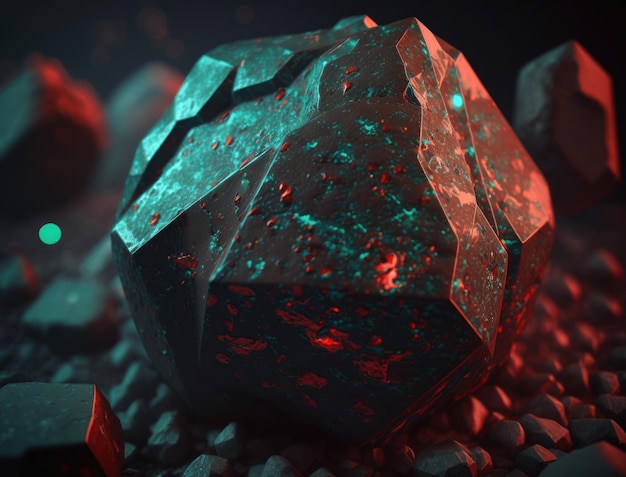The image depicts a diverse collection of pebbles scattered across the ground. Among them, some exhibit a reddish hue, while others are dark gray or black. In the background, a few larger stones with pointed tops are distinctly red. Additionally, a small green circle stands out amidst the pebbles. Notably, there is a particularly large stone, possibly a gemstone, positioned centrally in the image. This stone is predominantly black, adorned with red and green specks, and features a green circle upon its surface. It boasts a smooth texture and rises in multiple points, giving it a unique and striking appearance.